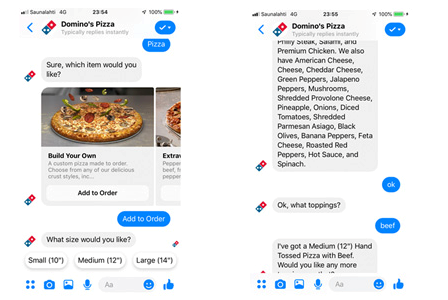In the image, you see a smartphone screen displaying a conversation between a user and Domino's Pizza, identified by Domino's logo and the contact name "Domino's Pizza" at the top. Below the title, in small grey letters, it notes, "typically replies instantly."

The conversation unfolds over two screenshots:

**Screenshot 1:**
- The user sends a message in a blue bubble that says, "Pizza."
- Domino's replies in a grey bubble, "Sir, what item would you like?" followed by an image of a pizza with various toppings like green peppers and pepperoni being added to it.
- Below the image, there's a grey box labeled "Build Your Own," with a description in smaller grey text, "A custom pizza made to order; choose from any of our delicious crust styles, etc."
- Below this box, a white button labeled "Add to Order" is visible. A partially cut-off button next to it suggests another option, "Extra" something, with a cropped pizza image above it.
- The user replies, "Add to order," in a blue bubble.
- Domino's asks, "What size would you like?" presenting three buttons: "Small (10 inches)," "Medium (12 inches)," and "Large (14 inches)."
- The bottom of the screen shows familiar messaging icons: menu (four blue dots), camera, attachment, microphone, text box with an emoji icon, and thumbs up.

**Screenshot 2:**
- Starts with Domino's listing potential toppings: Philly steak, sausage, premium chicken, American cheese, cheddar cheese, green peppers, jalapeno peppers, mushrooms, shredded provolone cheese, pineapple, onions, diced tomatoes, shredded parmesan, asiago, black olives, banana peppers, feta cheese, roasted red peppers, hot sauce, and spinach.
- The user replies, "Okay."
- Domino's responds, "Okay, what toppings?"
- The user answers, "Beef."
- Domino's confirms, "I've got a Medium (12 inch) pizza with beef. Would you like any more?" This message cuts off at the bottom.
- The bottom of this screen mirrors the same message icons as the first screenshot.
- The top of both screenshots displays a standard smartphone status bar showing 4G signal, the time (23:50 in the first screenshot and 23:55 in the second), a location icon, and a 100% battery charge indicator with a green battery icon.

The screenshots are clear, showing a smooth, step-by-step process of ordering a customized pizza from Domino's through a messaging interface.